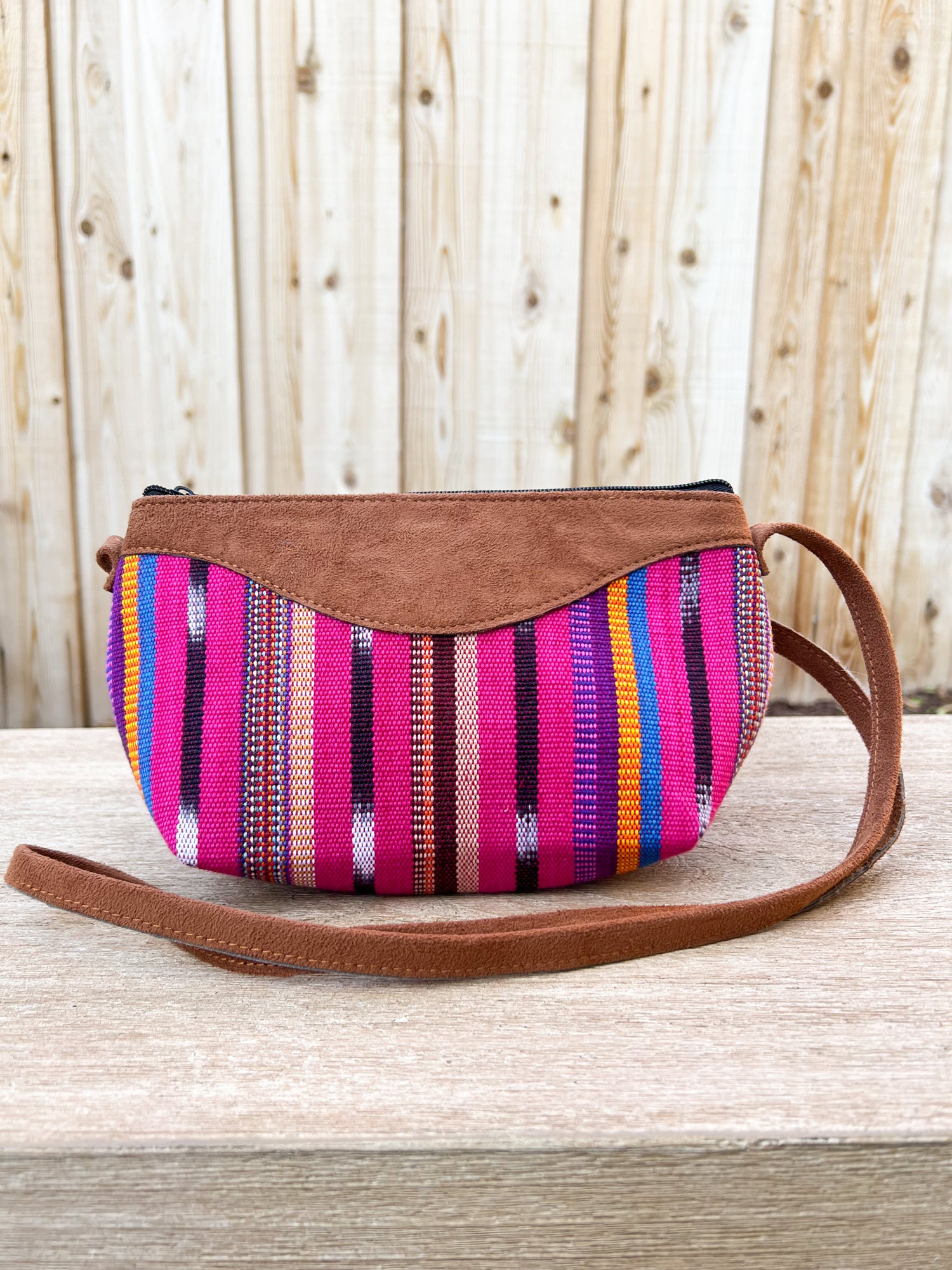The color photograph features a unique handbag set on a beige-gray wooden bench outdoors, with a backdrop of a driftwood-colored plank fence. The fence showcases a mix of white and dark brown grain with some knots, enhancing the rustic outdoor scene. The purse has a distinctive design: the body is constructed from fabric showcasing vibrant vertical stripes in shades of purple, yellow, blue, pink, cream, black, and white. The top trim and the long, slender strap are crafted from brown suede, with the strap featuring yellow stitching which curves around to the front. The bold, colorful stripes stand out strikingly against the brown suede, giving the bag a handmade, artisanal appearance.